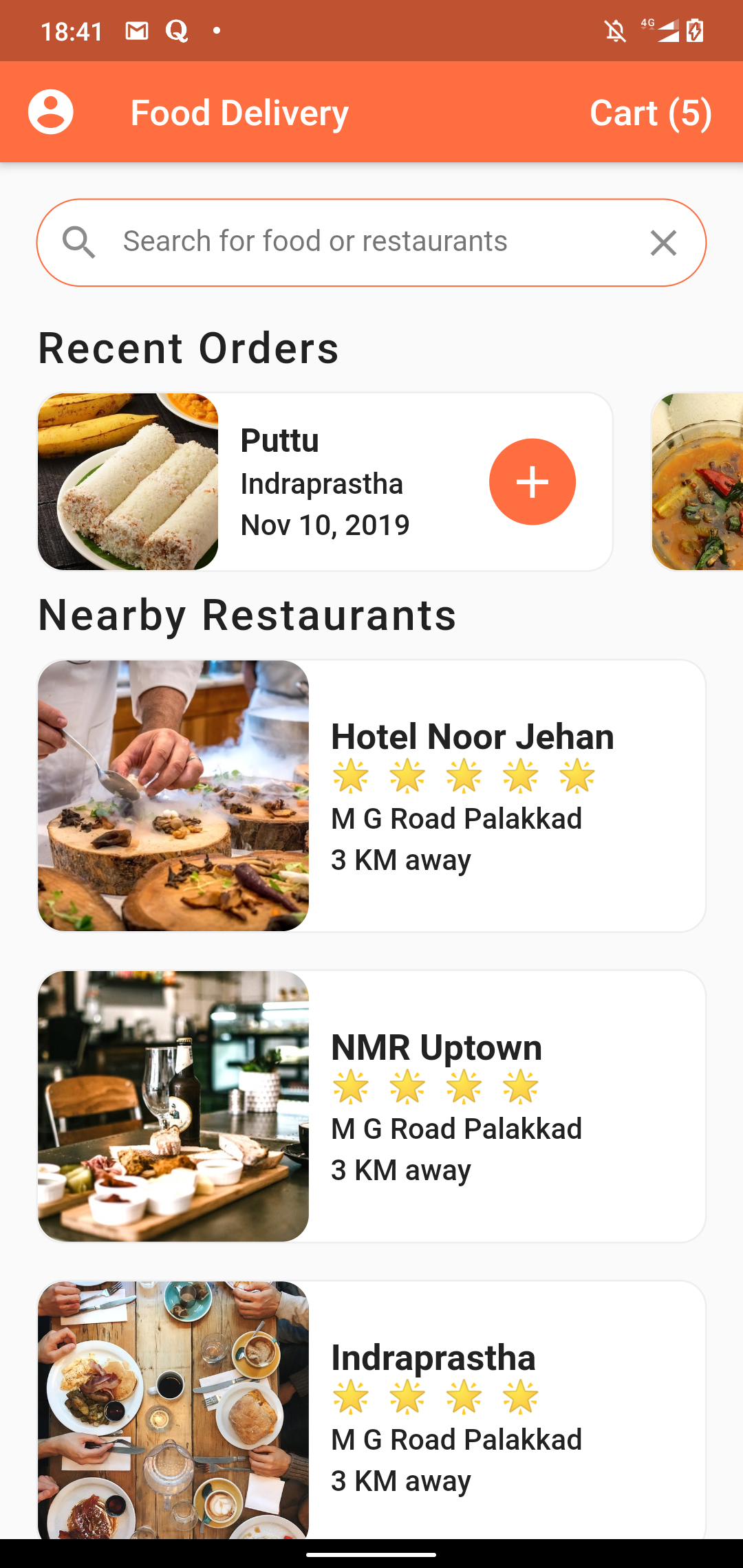The screenshot displays a smartphone interface from a food delivery app with the time highlighted as 18:41. At the top, the status bar indicates "Food Delivery" with a cart icon showing five items. Below this, the interface features a gray background, a search bar symbolized by a magnifying glass and an 'X' icon, with the placeholder text "Search for food or restaurants."

Beneath the search bar, the section titled "Recent Orders" displays an image of a plate of burritos alongside the text "Putu Indra Presta, November 10th, 2019." A red oval icon featuring a white plus sign appears next to this order.

Further down, the app showcases a "Nearby Restaurants" section with a list of eateries, each accompanied by a thumbnail image resembling a generic stock photo of a kitchen. The top entry is "Hotel Nord Johan," rated five stars, located at MG Road, Palakkad, 3 km away. Following it is "NMR Uptown" located on MG Road, Palakkad, 3 km away. The final listed restaurant is "Indra Presta," also situated on MG Road, 3 km from the current location.